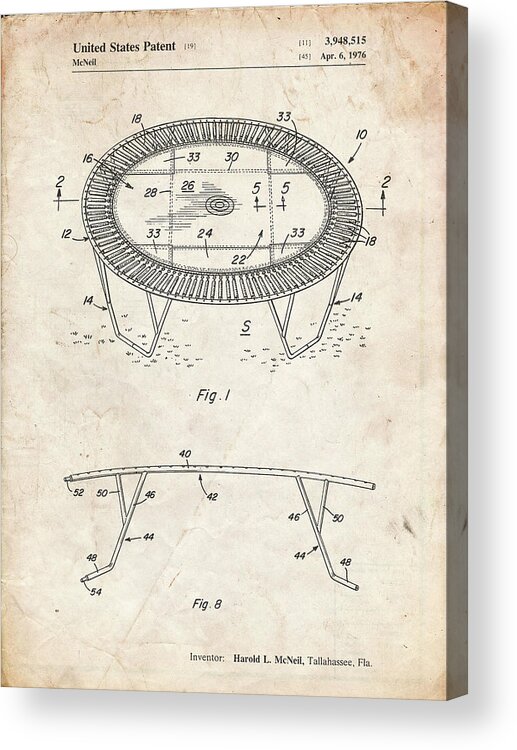This is an older drawing of a patent for a trampoline, dating back to April 6, 1976. The image shows a detailed diagram with two main views. At the top, it says "United States Patent" followed by "McNeil" and the patent number "3,948,515". The drawing is a bit aged, with the white background now turned brownish. The trampoline depicted in the drawing features a stitched-together canvas in the center, encircled by springs attached to a metal frame with metal legs extending to the ground. The upper portion of the drawing is labeled "Figure 1," showing a top view, while the bottom portion labeled "Figure 8" displays a side view, indicating different numbered components of the trampoline. The names "Inventor Harold L. McNeil" and "Tallahassee, Florida" are noted at the bottom.